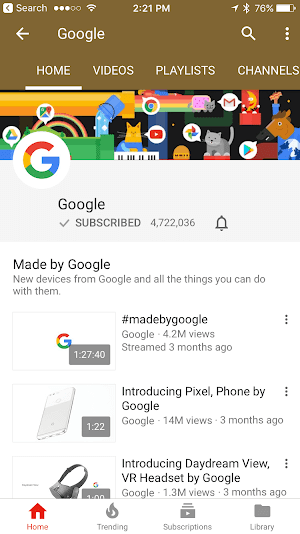This is a detailed description of a smartphone screenshot, showcasing a Google search interface:

At the top of the screenshot, there is a brown banner with a navigation bar. The navigation bar includes a search icon and a left-facing arrow situated at the very top. Adjacent to these elements are five dot indicators, with three dots on the left highlighted in white, signifying the current page. Following this, there is a Wi-Fi icon indicating a good signal, the current time displayed as 2:21 PM in the center, and, on the far right, a send icon, a Bluetooth icon, and a battery icon showing a 76% charge.

Beneath the banner, there is another left-facing arrow, subsequent to which is the word "Google" aligned to the right, followed by a search icon, and three vertical dots representing additional options.

Below these navigation elements are four tabs: Home (the current tab), Videos, Playlists, and Channels. Within the Home tab, various familiar Google logos appear—Google Play Store, Gmail, YouTube, and Google Docs—interspersed with cartoonish images of a cat, a horse, and a crescent moon, all interacting with these logos.

Further down, there is a grey section labeled "Google," featuring a check mark, indicating a subscription status with a count of 4,722,036 subscribers, and a notification bell icon. Directly beneath, it states "Made by Google" with a brief description: "New devices from Google and all things you can do with them."

Following this section, three video thumbnails are displayed: 
1. The first video, titled "Made by Google" with a duration of 1 hour, 27 minutes, and 40 seconds.
2. The second video, titled "Introducing Pixel phone by Google," lasting 1 minute and 22 seconds.
3. The third video is titled "Introducing Daydream View, VR headset by Google," with a duration of 1 minute.

At the bottom border of the screenshot, there is a navigation bar showing the Home tab (current view), along with additional tabs for Trending, Subscriptions, and Library.